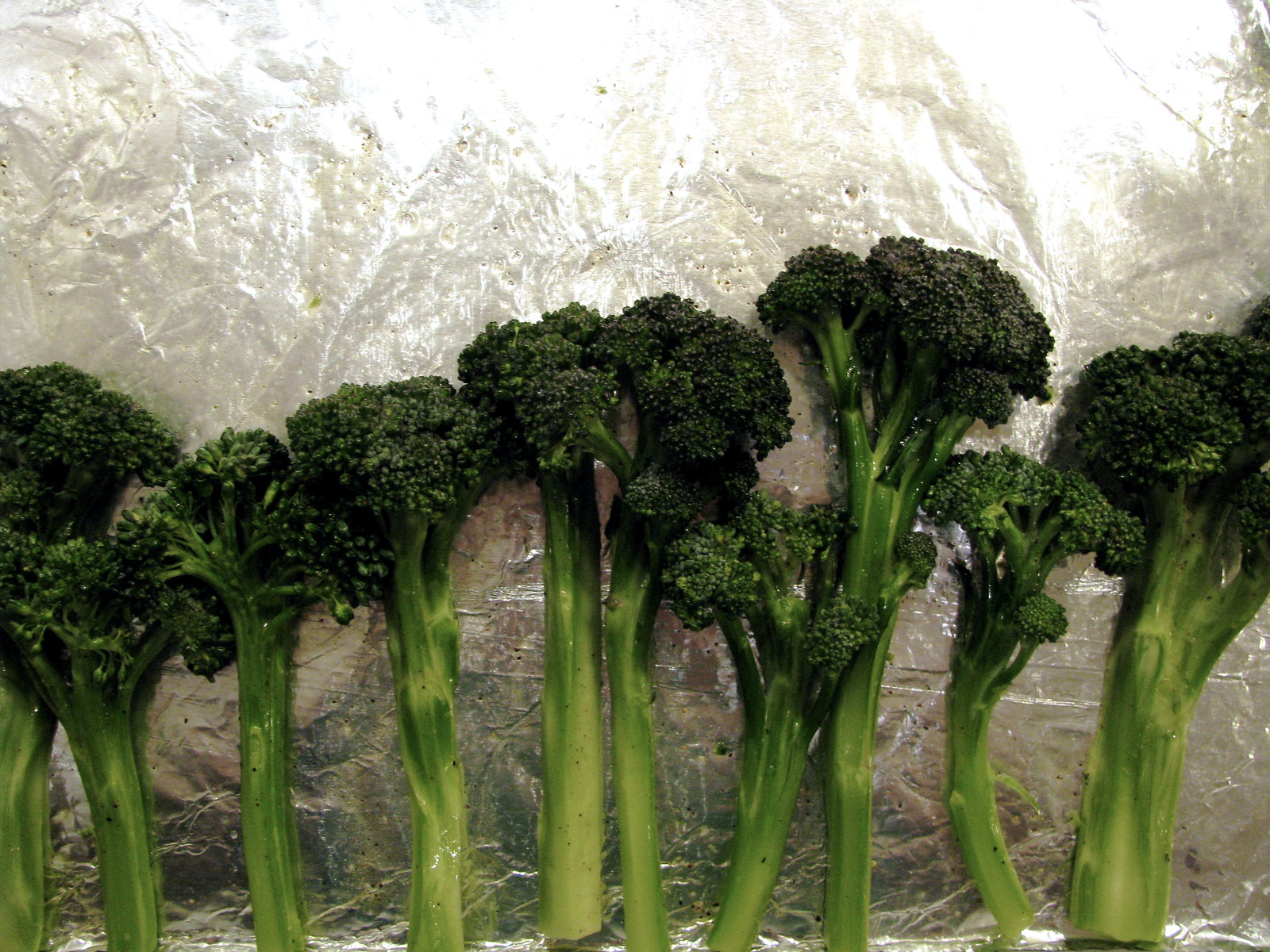This is a detailed photograph of ten roasted broccoli florets arranged on a sheet of aluminum foil. The foil, slightly bent up at the edges like a wall, creates an interesting silvery backdrop with reflections from a light source pointing directly at it. The broccoli pieces vary in size and shape, with the shortest ones on the left and gradually increasing in height towards the right. In the middle, there are two smaller broccoli pieces. The stalks are predominantly light green with bushy, dark green heads, indicating they've been cooked, likely with a coating of oil given their glistening appearance. The scene gives a charming semblance of tiny green trees or figures standing and mingling against the textured, shiny surface of the aluminum foil.